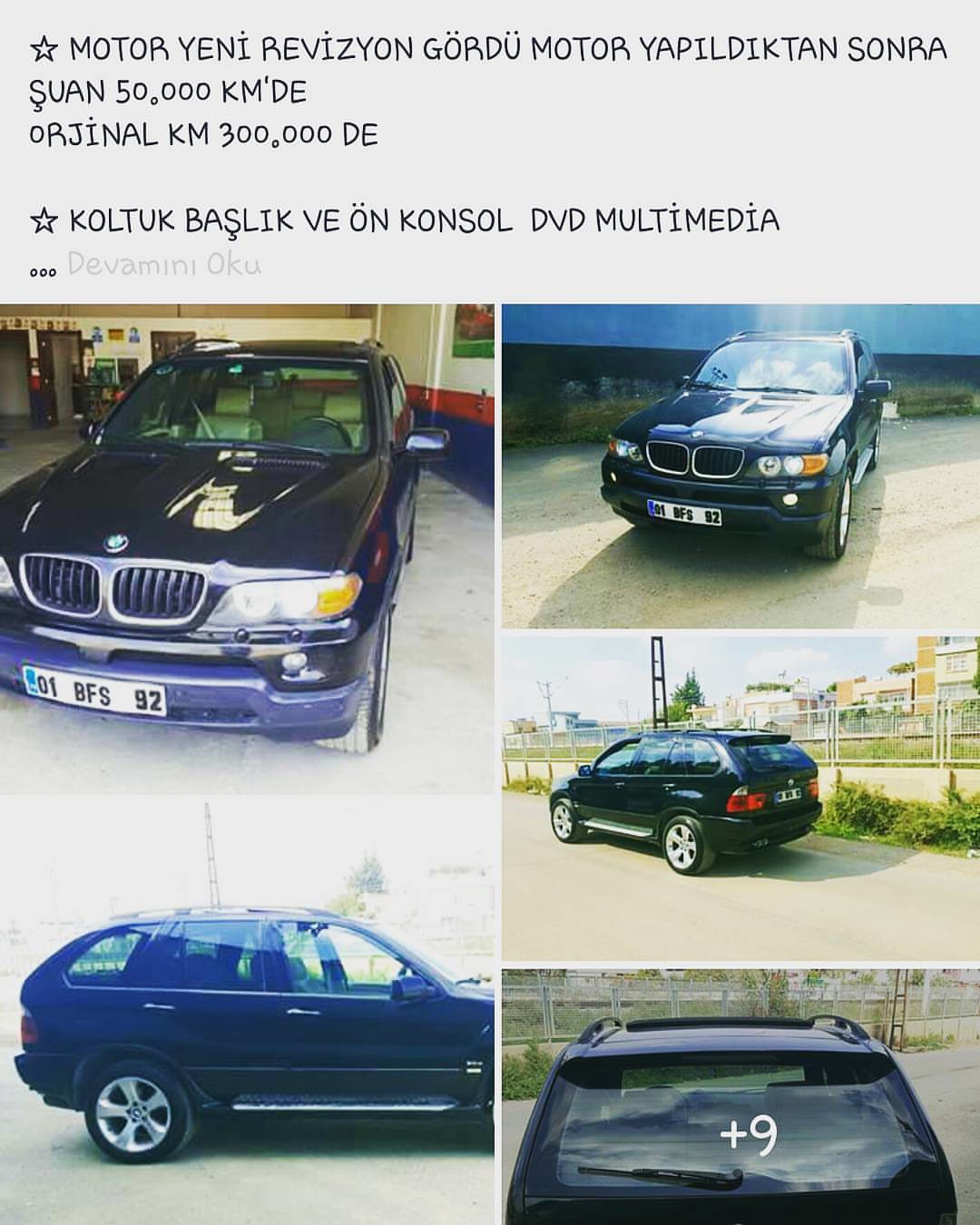The image appears to be an advertisement for a BMW SUV. The ad features five distinct photos of the vehicle arranged in two columns. The top of the ad showcases a horizontal gray bar with black text in a foreign language. The text likely provides details about the car's condition and specifications. 

The first line of the text includes the word "MOTOR" twice, along with "YENI REVIZYON GORDU," which suggests the engine has had a recent revision. Another line mentions "S-U-A-N 50 K-M'D-E," potentially indicating the current kilometer reading or another metric related to the vehicle's mileage. The text also includes "ORJINAL K-M 300,000 D-E," which might relate to the car's total mileage. Another part of the text mentions features like "KOLTUK BASLIK VE ON KONSOL DVD MULTIMEDIA," hinting at advanced multimedia features within the car.

The photos show the BMW SUV from different angles. The top left image captures the front view of the car inside a garage, displaying a closer look at the grille, hood, and windshield with a visible license plate. Below that, another image shows a side view of the passenger side, highlighting the wheels and trim. On the top right, the SUV is photographed from the front outside on a sunny day, positioned on a road with a wall visible in the background. Beneath this, a rear-side image of the car showcases it on a bright day with buildings around. The bottom right photo presents the back of the SUV with "plus nine" written on the rear window, implying there are additional images available.

The photographs collectively depict a dark blue BMW SUV, showcasing its exterior from various perspectives to thoroughly represent the car's condition and appeal.